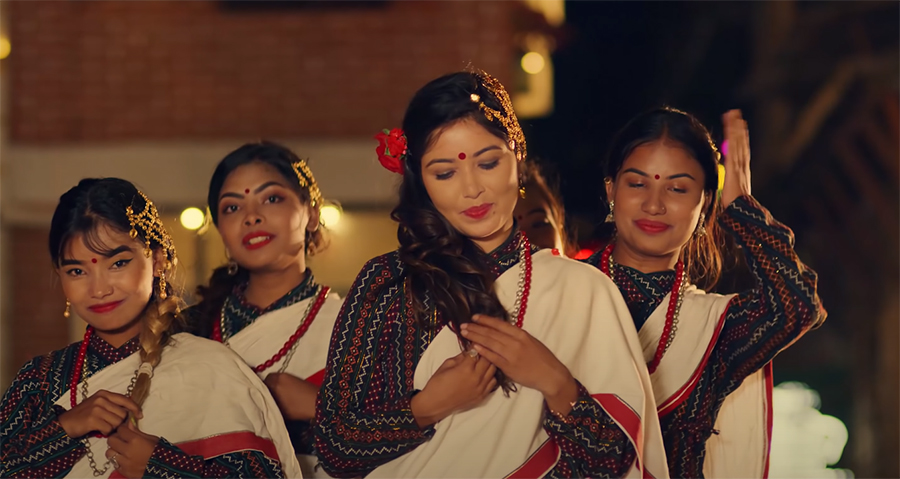The image depicts four women, likely of Southeast Asian or Indian heritage, adorned with traditional attire and bindis (red dots) between their eyebrows, suggesting a cultural or religious significance. Each woman is dressed in a zigzag blue, white, and red patterned long-sleeved garment, complemented by a white sash with red-outlined borders draped over one shoulder. They have dark hair styled in braids, embellished with gold lace hair accessories, and a red rose in the hair of the woman positioned slightly in front. With gentle smiles and expressive makeup including red lipstick and eyeshadow, their poses imply they are either dancing or are about to commence a traditional dance. The background is blurred, emphasizing the focus on their garments and expressions in the nighttime setting.